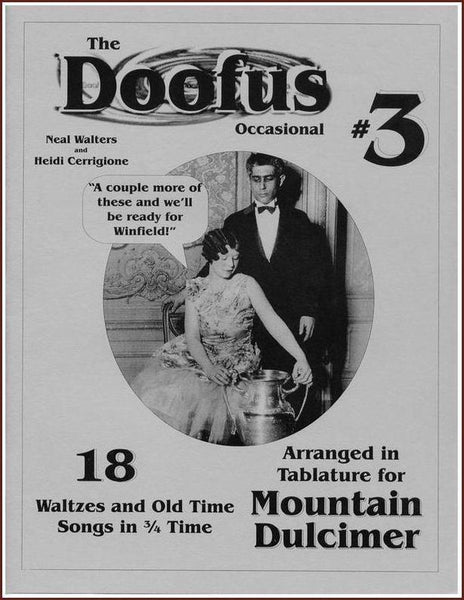The image depicted in the booklet or poster features a vintage black and white photograph framed in a circular border, showcasing a man and a woman dressed in early 20th-century fashion. The woman, seated in a chair, is sporting wavy finger waves and a sleeveless printed gown reminiscent of the 1920s-1930s style. She is holding what appears to be a silver two-handled vase or trophy. Standing behind her is a man in a black tuxedo with a black tie and white shirt, his hand resting on the back of her chair. The image is overlaid with several text elements: the title "The Doofus Occasional Number 3" across the top, followed by the names "Neil Walters and Heidi Seraglioni." A speech bubble next to the woman reads, "A couple more of these and we'll be ready for Winfield." Additional text at the bottom left advertises "18 waltzes and old-time songs in three-quarter time," while the bottom right indicates that the content is "arranged in tablature for Mountain Dulcimer." The overall presentation suggests that this is a promotional poster or cover for a musical booklet, emphasizing old-time music and waltzes.